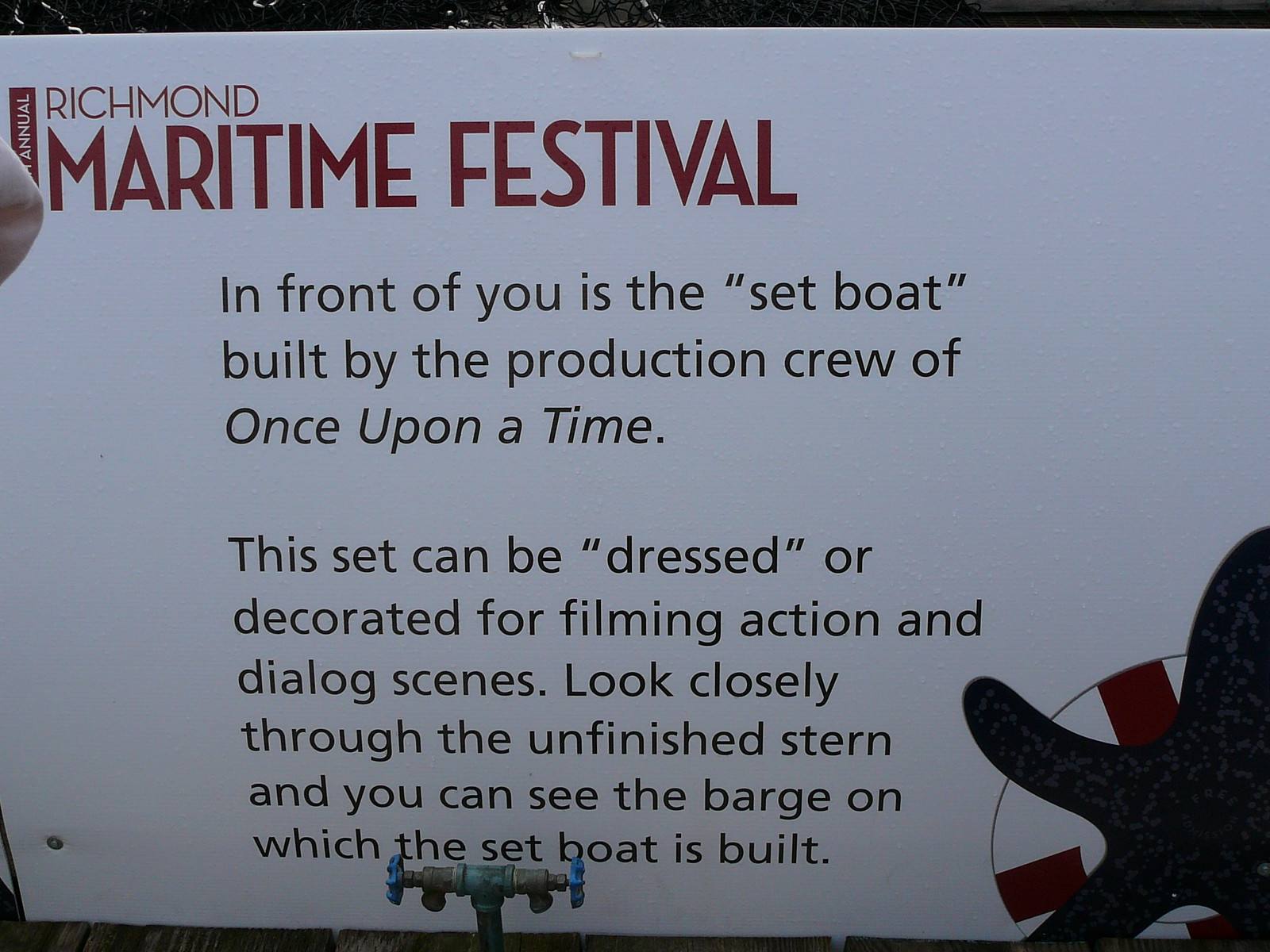The photograph showcases a somewhat dark and shadowed rectangular sign that appears to be outdoors, with tree branches peeking in at the top. The sign reads "Annual Richmond Maritime Festival" in prominent lettering at the top, possibly including a number such as "30th" before "Annual." Below, it states, "In front of you is the set boat, built by the production crew of Once Upon a Time. This set can be dressed or decorated for filming action and dialogue scenes. Look closely through the unfinished stern and you can see the barge on which the set boat is built." The foreground features a water spigot with a T-shaped pipe and two hose nozzles sticking out, creating an odd juxtaposition with the sign. Partial elements of a starfish or octopus outline and a life preserver appear towards the lower corners of the image. Overall, the scene is dim and subdued, obscuring some details.